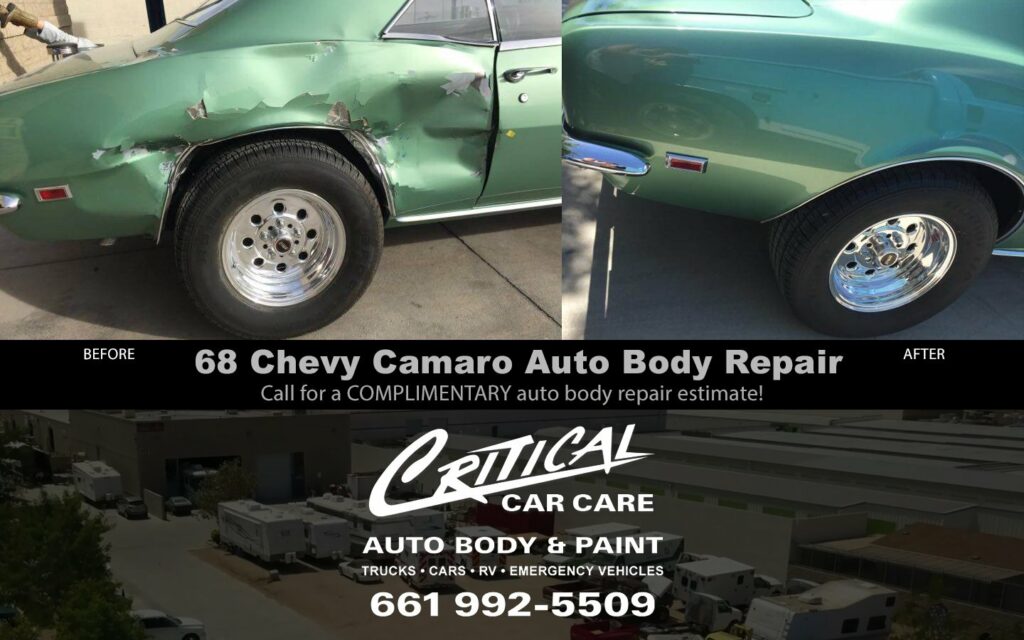The advertisement for Critical Car Care, Auto Body, and Paint showcases a meticulous auto repair service. The top portion features a 1968 Chevy Camaro in a darker mint green shade with noticeable damage to its rear right quarter panel and door, particularly above the wheel, where the area is significantly collapsed. To the right, the car is presented in its restored state with buffed and shined paint, and all dents, particularly around the wheel area, expertly repaired to look as good as new. The ad emphasizes their service offerings for trucks, cars, RVs, and emergency vehicles, and includes a call-to-action for a complimentary repair estimate. The company's logo and contact number, 661-992-5509, are clearly displayed over a darkened backdrop of the body shop's location, reinforcing their brand and expertise in auto body repair.